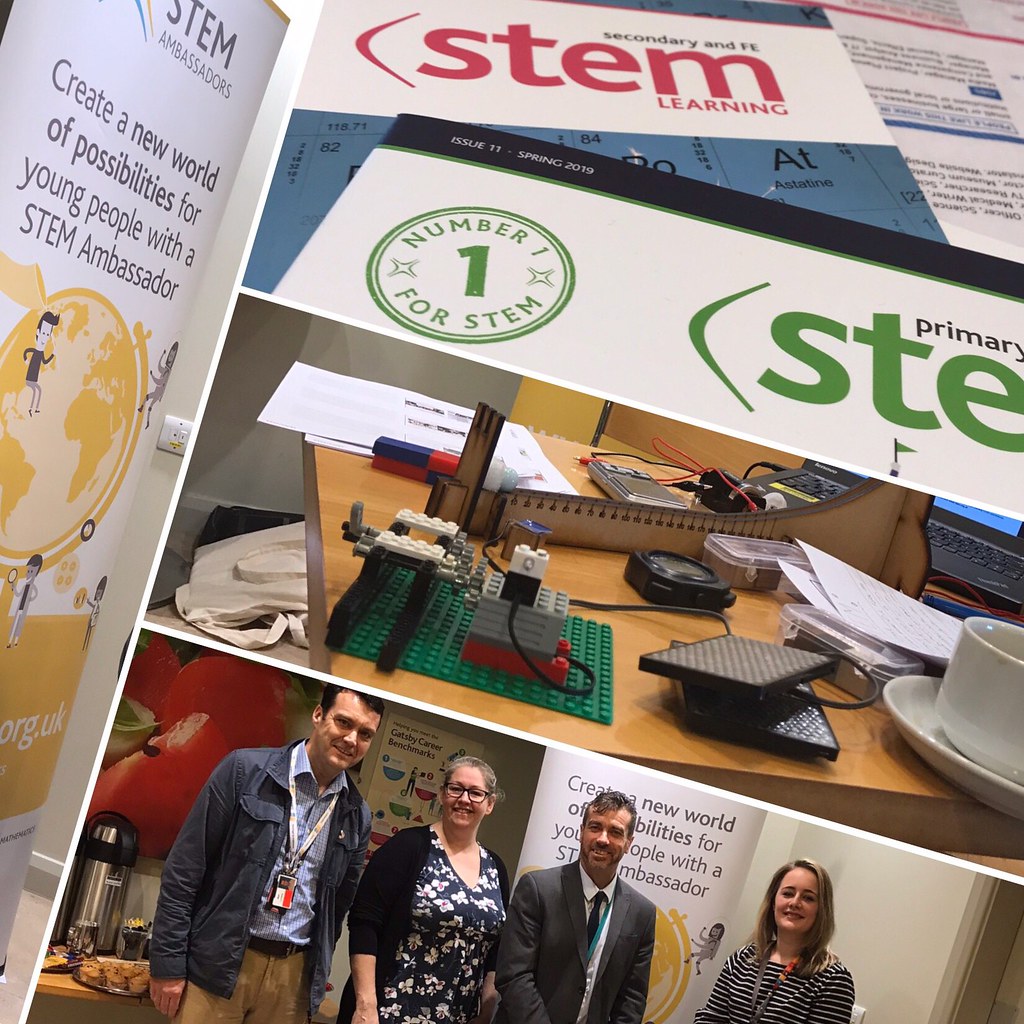The image is a detailed poster promoting STEM learning and featuring STEM ambassadors. At the top, "STEM Learning" is prominently displayed in red letters against a white background. Just below, it says "STEM ambassadors" in bold dark print followed by the inspiring slogan "Create a new world of possibilities for young people with a STEM ambassador." To the left, there's a gold circular globe illustration, while the center is dominated by a large green circle with a number '1' and the phrase "Number one for STEM" written above it. To the right, a partially visible logo reads "STE" above "primary," cut off by the border of the image.

In the lower section of the image, there are four individuals standing in front of a billboard reiterating the slogan. From left to right: the first man wears a blue jacket, brown shirt, and a lanyard; next to him, a woman dons a blue and white print dress with a black sweater; the second man is in a gray suit coat and dark tie; and the last woman wears a black and white striped dress, brownish hair cascading over her front. Behind them, an image of computer interiors and a white cup on a saucer are visible, suggesting an environment rich in STEM activities. There are scattered signs and flyers, including depictions of young people and a mascot, creating a vibrant and engaging scene reflective of a STEM-themed event or convention.